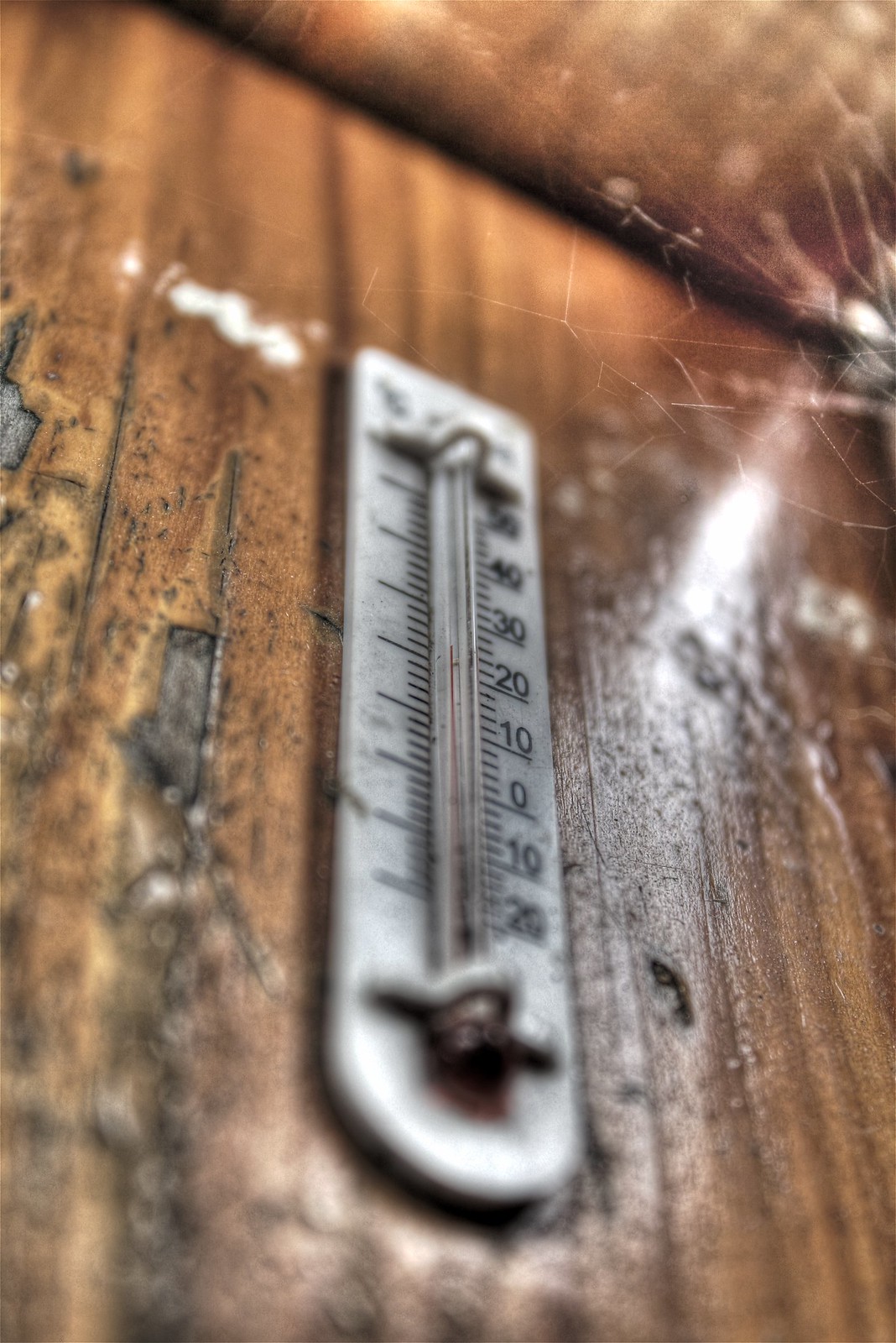The image depicts an old-fashioned thermometer mounted on a weathered, wooden wall, which seems to be part of either a neglected house, a barn, or an outbuilding. The wall surrounding the thermometer is marked with what appears to be mold or dirt, giving it a grimy look. The wood itself is aged, punctuated with pits and grayish marks, making it difficult to distinguish between dirt and natural wear. In the upper right corner of the image, a faint spider web can be seen, hinting at the area’s disuse.

The thermometer has a rectangular shape with a rounded bottom and squared-off top. The Fahrenheit scale is clearly marked on the right side, with numbers descending from 50°F down to -20°F, each separated by a series of small dash marks. The red liquid inside the thermometer, likely mercury or a similar substance, is visible. The left side of the thermometer is devoid of numbers, containing only lines corresponding to the Fahrenheit measurements, suggesting that it might typically display Celsius.

The wall itself is primarily brown with patches of darker colors, either from dirt or natural wood aging. Additionally, a subtle stream of sunlight illuminates the scene, adding an element of contrast to the overall dark and dingy appearance.